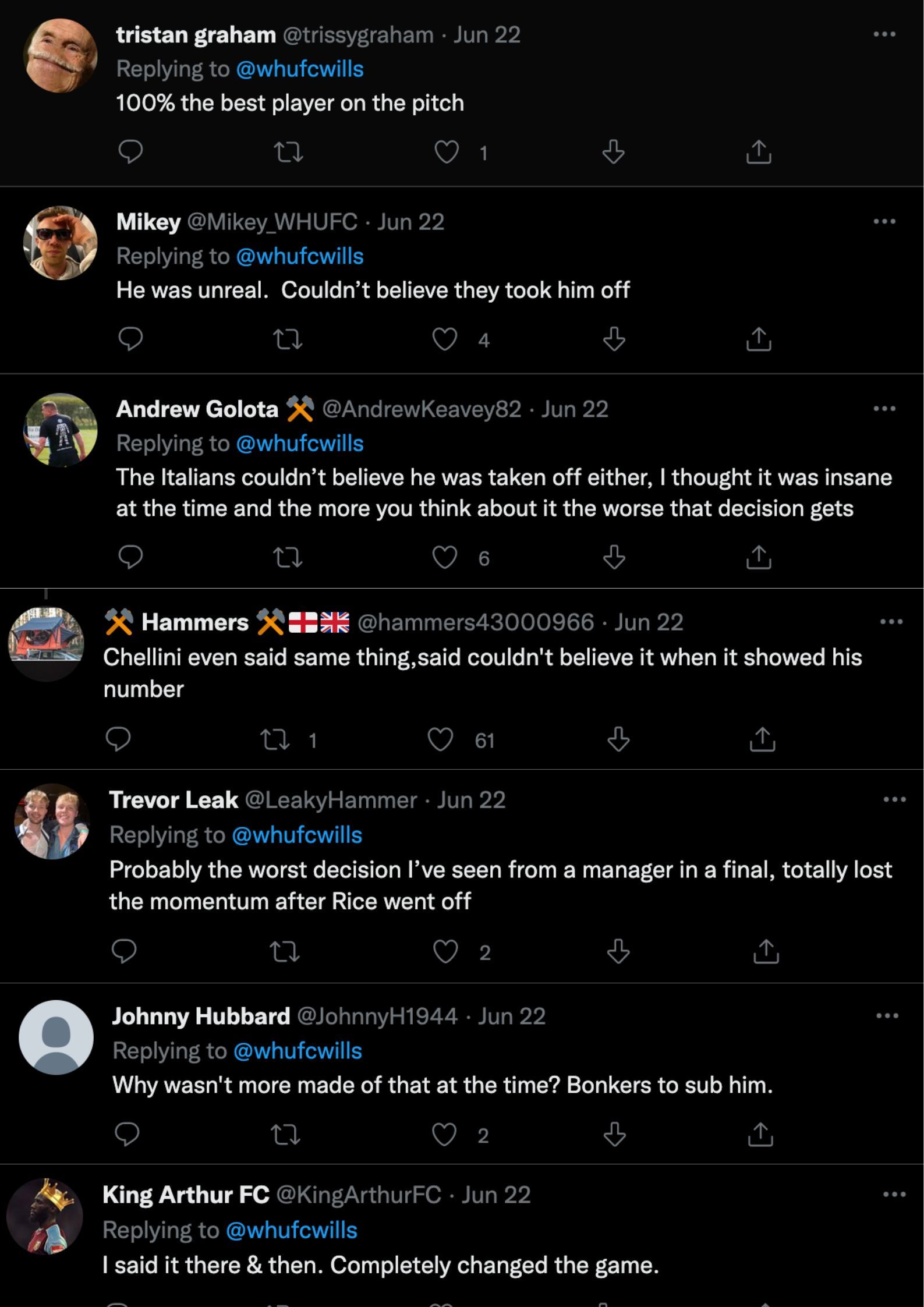### Social Media Reactions to a Key Player Substitution

In this image, we see several strips of a conversation, all set against a black background. The text appears in varying colors – white, gray, and blue. The dialogue centers around a controversial substitution during a football match on June 22.

1. **Tristan Graham (@TristanGraham)**
   - **Replying to @whufcwills**
   - This is 100% the best player on the pitch.

2. **Mikey (@whufc)**
   - **Replying to @whufcwills**
   - He was unreal. Couldn't believe they took him off.

3. **Andrew Golota (@AndrewKV82)**
   - **Replying to @whufcwills**
   - The Italians couldn't believe he was taken off either. I thought it was insane at the time, and the more you think about it, the worse the decision gets.

4. **Hammers (@hammers43000966)**
   - **Replying to @whufcwills**
   - Ch Lli and I even said the same. He said he couldn't believe it when they showed his number.

5. **Trevor Leak (leaky_hammer)**
   - **Replying to @whufcwills**

The overall sentiment in these reactions is disbelief and frustration over the substitution, highlighting the perceived impact and importance of the player who was taken off the pitch.